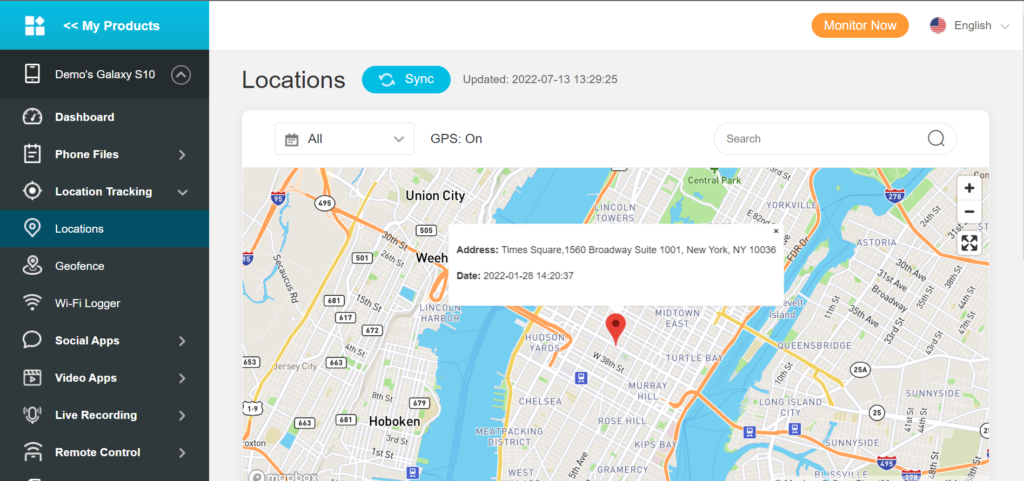A detailed depiction of a location tracking interface:

The image portrays a sleek and sophisticated location map interface, primarily set against a deep black background accentuated by vibrant turquoise and light blue highlights. Various categories are neatly listed in white text along the side, including "My Products," "Demo Galaxy S10," "Dashboard," "Phone Files," "Location Tracking," "Locations," "Geofence," "WiFi Logger," "Social Apps," "Video Apps," "Live Recording," and "Remote Control." Among these, "My Products" and "Locations" are distinctly highlighted in shades of blue and turquoise.

At the heart of the interface lies a detailed, interactive map displaying various locations. A prominent blue "Sync" button invites users to update the data, with the map's last update recorded on July 13, 2022, at 13:29:25. A noteworthy feature is located in the top right corner, where an orange "Monitor Now" button and a language selector (denoted by the word "English" alongside a flag icon) can be seen.

The map crucially marks an address in Times Square: 1560 Broadway Street, 1001 New York, New York, 10036. This specific location was recorded on January 28, 2022, at 15:20:37, indicated by a bold red marker pinpointing the exact spot. The map also offers a comprehensive view of the city's layout, enhanced by an operational GPS. Users can easily search for further details using a search button symbolized by a magnifying glass.